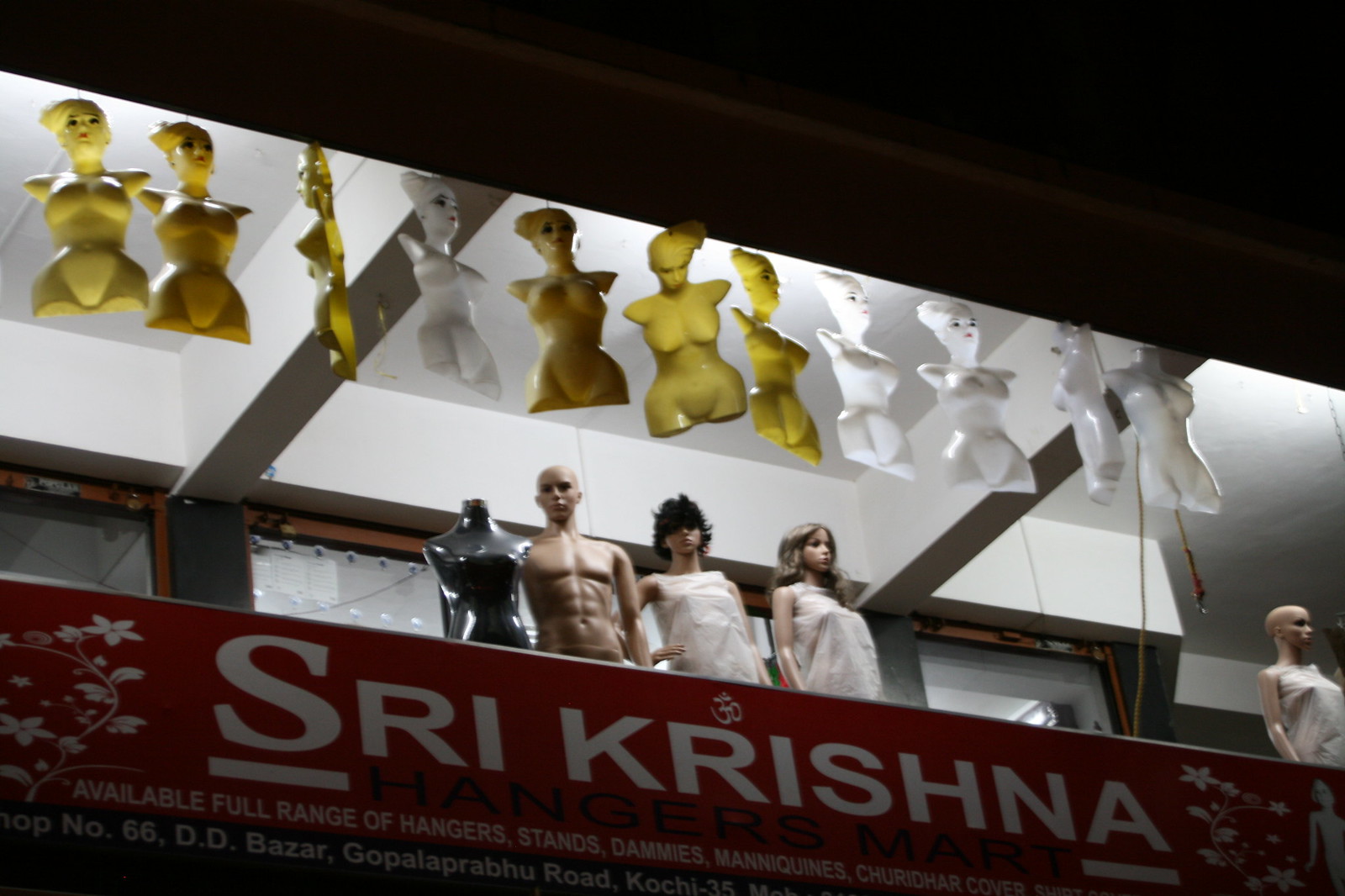The image depicts a storefront display showcasing a variety of mannequins arranged on multiple levels. Dominating the bottom of the scene is a bold red banner with white lettering that reads "Sri Krishna." A range of mannequins is situated above this banner, starting with a headless, shiny gray mannequin on the far left, standing directly atop the banner. Next to it, a male mannequin is visible, characterized by its bald head and lack of clothing. To its right, there is a female mannequin with short dark hair adorned in a white smock. Adjacent to her is another female mannequin with long blonde hair, also dressed in a white smock. On the far right, another female mannequin, bald and donning a dress, stands with one arm by its side.

Suspended above this lower row of mannequins are 11 half-bust mannequins, featuring torsos and heads of women but lacking arms and lower bodies. These mannequins are colored in shades of yellow and white, providing a stark contrast against the white walls and brightly lit backdrop of the storefront. Windows behind the display further suggest this is part of a mannequin maker's shop, offering a view into the store's interior and backing up the commercial nature of the setting. The overall arrangement creates a striking visual narrative of the diverse forms and designs of mannequins available at this store.